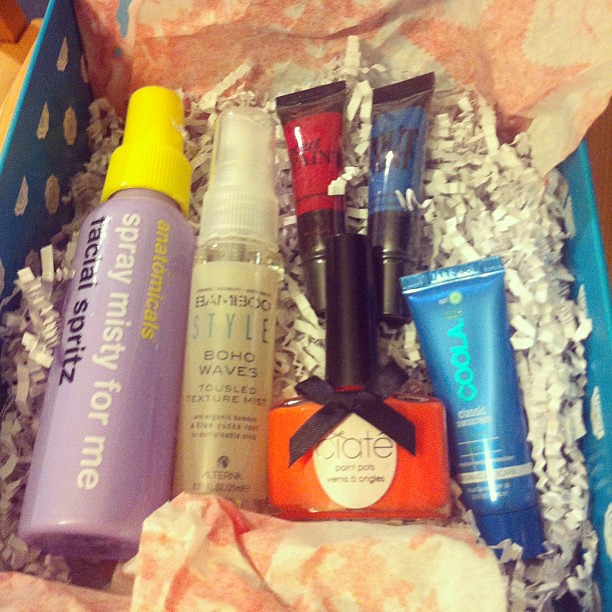The image features a square gift basket filled with a variety of women's beauty products. The basket itself has sides that are bright blue with white polka dots, visible at the top left corner and along the top right edge. The base of the basket is lined with light orange patterned tissue paper and filled with tiny white paper streamers.

Starting from the left, the first item is a tall, light purple bottle with a neon yellow cap that reads "Spray Misty For Me" in white font, indicating it is a facial spritz. Next to it is a slightly smaller clear bottle with a tan label that says "Bamboo Style Boho Waves Tousled Texture Mist," a product likely used for hair styling.

Further to the right is a bottle of orange nail polish adorned with a small black bow and a black lid. Above the nail polish, two small lip glosses can be seen. On the far right of the basket, there is a blue bottle, adding another element to the collection of beauty products. The basket is neatly wrapped in light orange patterned tissue paper, complementing the diverse array of items inside.